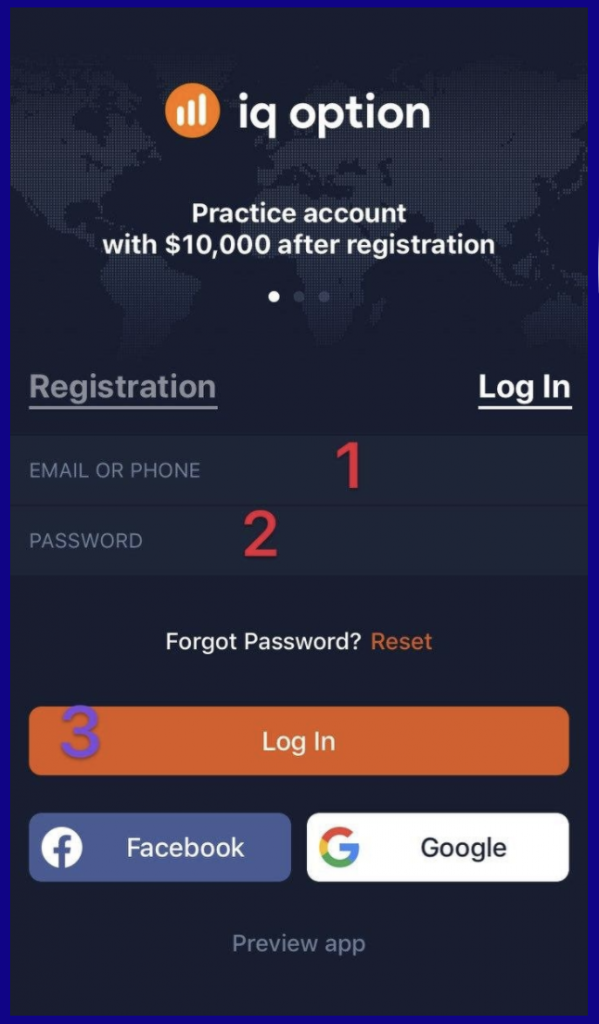The screenshot is from a mobile interface of IQ Option, a trading application. At the top, the image features a world map in a light bluish-gray tone set against a dark blue background. Prominently displayed in the center is the IQ Option logo: an orange circle housing three ascending bars from left to right. Adjacent to this logo, in lowercase lettering, it reads "IQ option."

Beneath the logo, the text states, "Practice account with $10,000 after registration," followed by three dot indicators, with the left dot highlighted in white. Below this section, there are options for "Registration" and "Login." The "Registration" button is rendered in a grayish-blue, while the "Login" button is in white and highlighted with an underline, indicating it is currently selected.

The next section offers two fields for user input: the first for "Email or phone," marked with a numerical "1," and the second for "Password," marked with a "2." Following these input fields, there's a typical "Forgot password?" text link, where the question "Forgot password?" is in plain text and the link "Reset" is in orange.

Finally, there’s a prominent "Login" button extending almost the full width of the app, colored in orange, and marked with a purple "3." Below the login button, there are two alternative login options. The left button is a light purple labeled "Facebook" with its logo on the left, and the right button is white labeled "Google" with its logo. At the bottom of the screen, there is an additional link that says "Preview app."